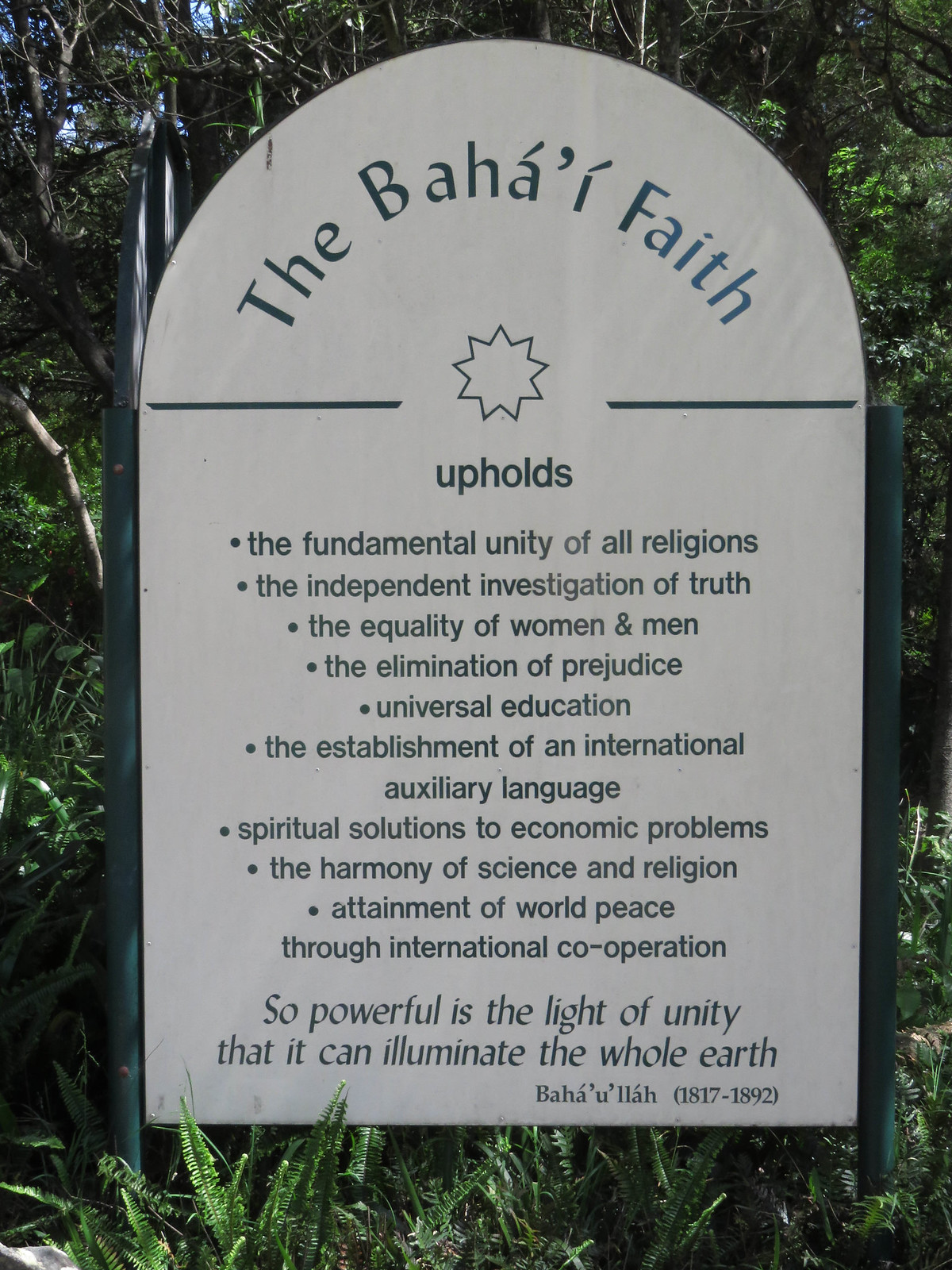This image captures an outdoor sign partially obscured by lush greenery, including ferns and other plants at its base, with trees visible in the distant background. The rectangular sign, which has a curved top and is held in place by metal poles, features prominent greenish-bluish aqua text. It begins with "The Baha'i Faith," followed by a star or explosion-like symbol. Below, the sign highlights the Baha'i Faith's key principles in bullet point format: the fundamental unity of all religions, the independent investigation of truth, the equality of women and men, the elimination of prejudice, universal education, the establishment of an international auxiliary language, spiritual solutions to economic problems, the harmony of science and religion, and the attainment of world peace through international cooperation. At the bottom of the sign, in a different font, it reads, "So powerful is the light of unity that it can illuminate the whole world. Baha'u'llah 1817-1892."